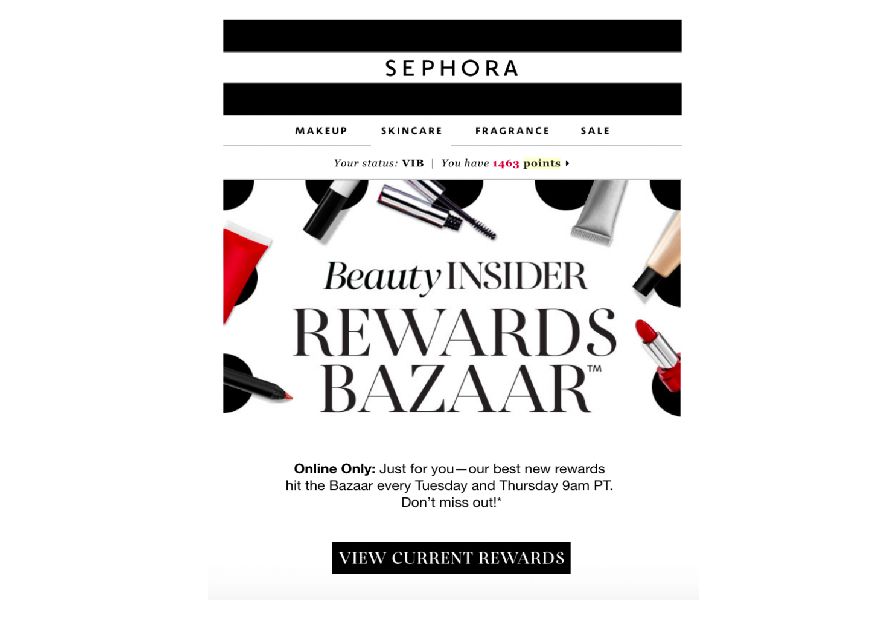The image, sourced from a Sephora website, prominently displays an interface focused on beauty and makeup offerings. At the top of the screen, there are three horizontal rectangles: a black one, a white one, and another black one, spanning across the width of the phone. Inside the central white rectangle, "SEPHORA" is written in bold, black, all-capital letters.

Beneath this banner, a secondary menu lists "Makeup," "Skin Care," "Fragrance," and "Sale" in black letters. Progressing further down, the screen shows the user's status as "VIB," indicating they have accumulated 1,463 points. The point count '1463' stands out in red, and the word "points" is subtly highlighted in yellow.

The next section features the "Beauty Insider" and "Rewards Bazaar," where 'Bazaar' is spelled out as B-A-Z-A-A-R. Below this, a message reads: "Online Only, just for you. For Best New Rewards, hit the Bazaar every Tuesday and Thursday, 9 a.m. PT."

At the bottom of the image, a final call to action states "Don't Miss Out," followed by a black box with the text "View Current Rewards" printed in white.